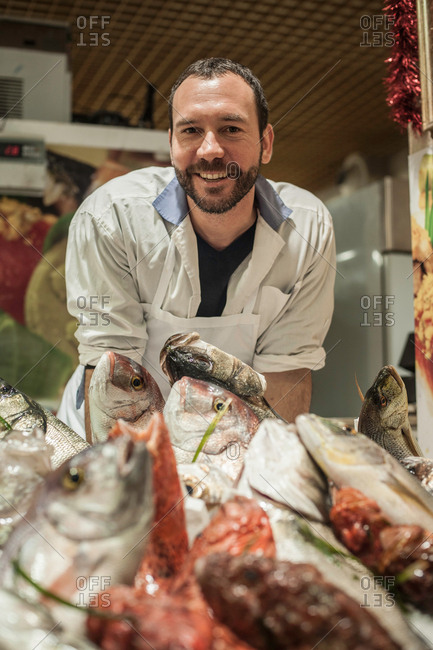This is a detailed portrait-oriented color photograph depicting a smiling Caucasian man working as a vendor in a fish market. He is dressed in a white apron over a cream-colored shirt with a gray collar. His appearance includes a dark beard and mustache, with thinning dark hair combed back. The man is standing behind a counter full of various fish parts, including cut-up heads, bodies, and insides, showcasing a range of sizes, shapes, and colors. The frozen fish pieces are stacked in front of him, indicating they are ready for sale.

In the background, the fish market environment is partially visible, featuring a white refrigerator on the right side, a wood trellis ceiling overhead, and other indistinct market elements on the left. The photograph employs a style of photographic representationalism, capturing the realism of the scene. Additionally, the image contains a watermark with the text "OFF13S" in several places. The vendor's cheerful demeanor and propped stance on the countertop convey a welcoming and approachable atmosphere in the bustling market setting.